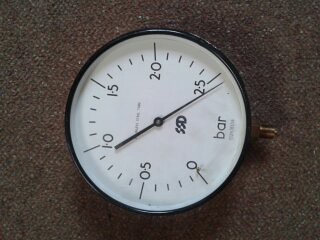The image depicts a small, square photograph featuring an object placed on a gray, carpet-like background. At the center, there is a compact, white, round dial mounted on a black base. Protruding from the right side of the base is a small metal nodule. The middle of the dial is covered with a glass surface, displaying a white face marked with numbers and dashes, resembling a thermometer or barometric pressure indicator. The scale on the dial starts at zero at the bottom and ascends to 25 at the top, with a fine, black pointer currently indicating the number 25. Just above the center of the dial, the letters "SSD" are printed in black font, while the word "bar" appears on the left side. The overall design suggests it is an indicator for measuring a specific parameter, though the exact purpose remains unclear.